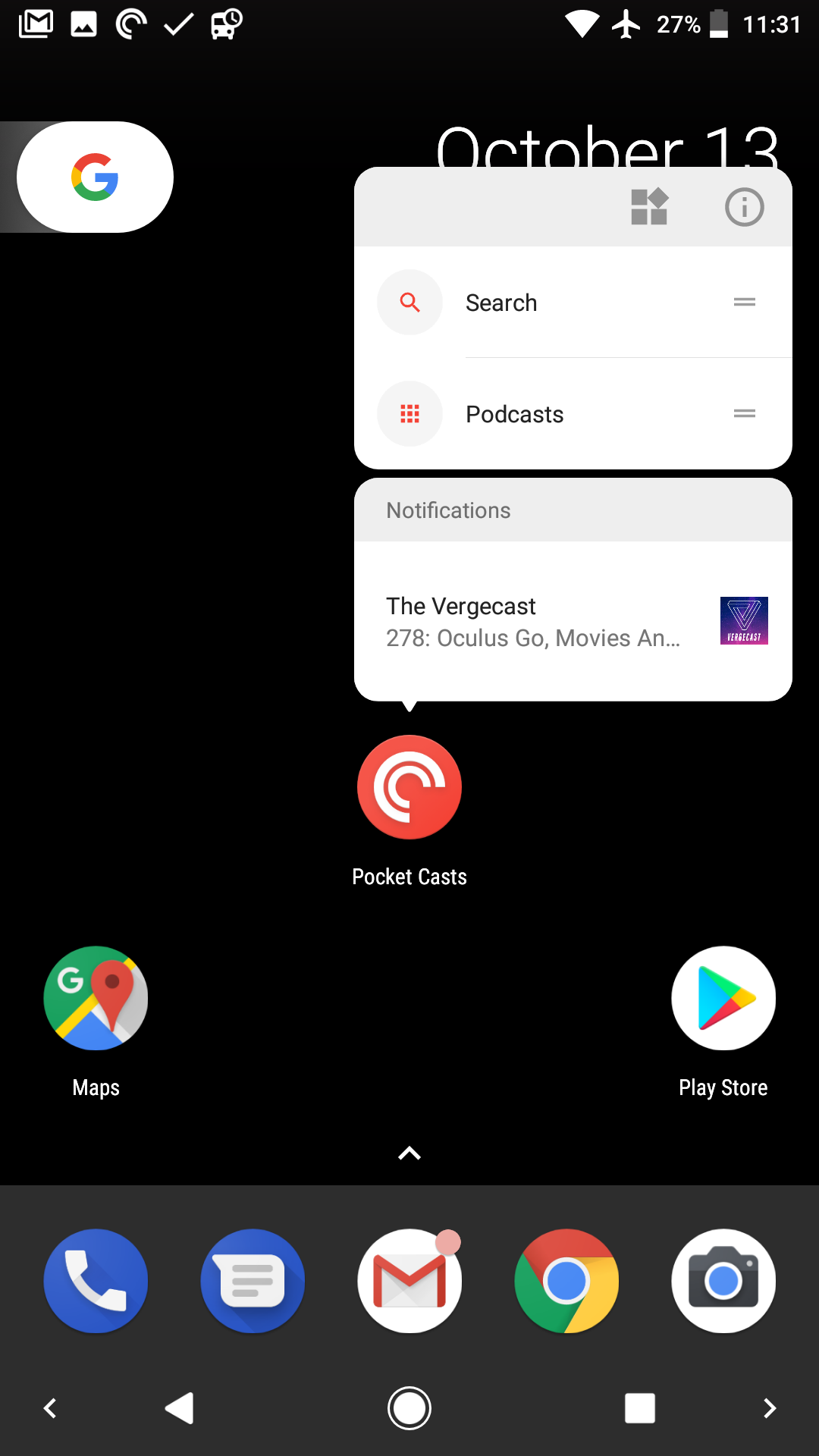A detailed description of the image depicted on a cell phone screen:

The cell phone screen shows the current time as 11:31, with a battery level at 27%, indicating about a quarter of the battery remaining. The phone is in airplane mode and has a strong connection signal. On the left side of the screen, there's an image that appears to be a bus, accompanied by a circle with a checkmark and three-quarters of a circle, representing some activity.

Further down, there's an icon for Gmail and another application that looks like a notes app. Dominating the center of the screen, there is a white circle with a multi-colored letter "G" representing Google. The date displayed is October 13th. Slightly above this, there is a pop-up search box with the word "podcasts."

Below the date, another notification box pops up, featuring "The Vergecast" with a title underneath that reads "Oculus company movies." This notification includes a small, purple and pink picture, and is topped with the podcast icon—a red circle containing a white play button.

To the right, there are icons for Maps, showing the classic map icon with a red pin, and the Play Store, represented by the Google triangle logo. At the very bottom of the screen, there are icons for the phone app, a notes app, Gmail (marked with a small circle), Google Chrome, and a large camera icon.